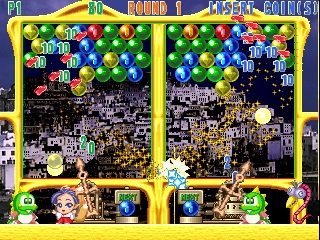The image is a vibrant, action-packed screenshot from a video game, indicative of a classic arcade setup. At the top-left corner, "P1" in green designates Player 1, who has accumulated 80 points. Centrally positioned at the top, the text indicates that the game is currently in "Round 1." On the top-right corner, "Insert Coins" is displayed in blue, likely prompting additional input for play.

The heart of the image features two sides reminiscent of an arcade game backdrop, bustling with colorful balloons in shades of yellow, green, red, and blue. The balloons stand against a detailed and busy background resembling an ancient city, potentially Greek, inferred from the architectural styles of the buildings.

Within the game area, two white square shapes can be seen. At the bottom of the screen, four distinct characters are engaged in shooting arrows upwards to pop the balloons. Among the characters, two resemble small dragons or Yoshis, one is a human figure, and the last appears to be a snake-like creature. The combination of the animated figures and the dynamic background creates a lively and captivating scene, echoing the traditional excitement of vintage arcade games.